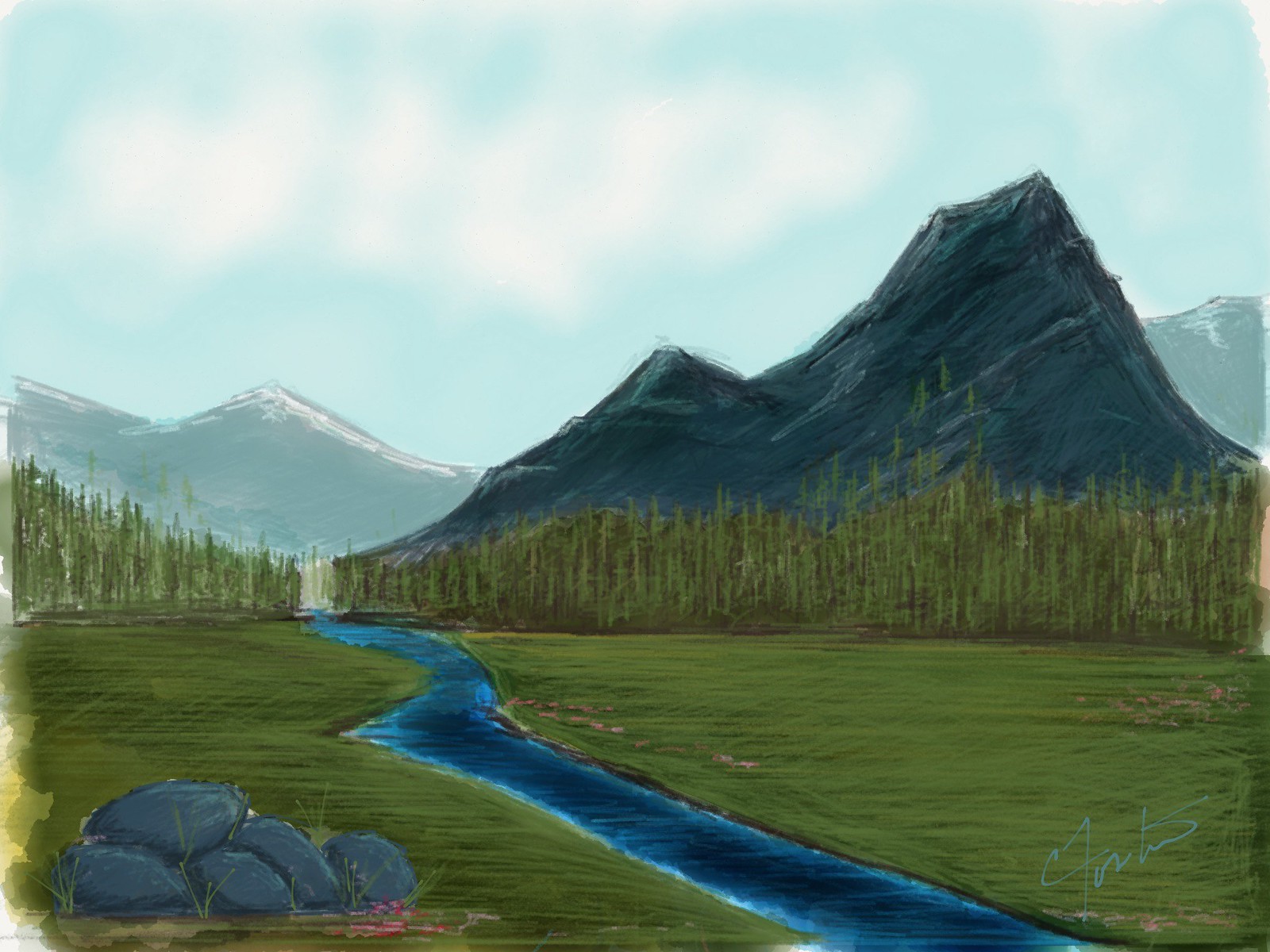A breathtaking square-shaped artwork captures a serene nature scene, exuding tranquility through its vivid depiction. Dominating the upper portion of the image, a sky painted in delicate shades of light blue and white is interspersed with soft, fluffy clouds. Below this peaceful expanse, towering mountains emerge, adding a magnificent sense of scale and grandeur to the piece. On the bottom left, rugged gray rocks anchor the scene, nestled amid lush green plants that breathe life into the composition. A crystal-clear stream meanders gracefully down the center of the artwork, flanked on either side by expansive fields of vibrant grass. The artist's initials, inscribed in delicate light blue cursive, are subtly placed in the bottom right corner, adding a personal touch to this exquisite embodiment of nature's beauty.